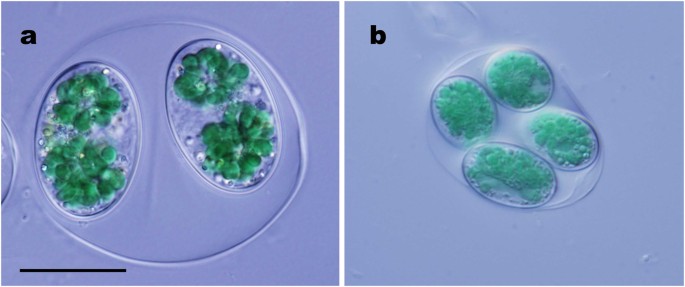This detailed image comprises two side-by-side photographs labeled A and B, taken under a microscope and separated by a small white space. Both images rest on a lavender or blue background. In photograph A on the left, two algae cells are visible within a droplet of water placed on a white sheet. Each cell features thin, transparent outlines and is filled with green droplets or dots. A partially cut-off cell appears to the left of these two. In photograph B on the right, a larger droplet contains a single clear circle housing four smaller cells, each filled with green bubbles, suggesting further cellular division. The overall layout of the image features a rectangular format with each section close to a square shape, highlighting the cell division process from two cells in A to four cells in B.